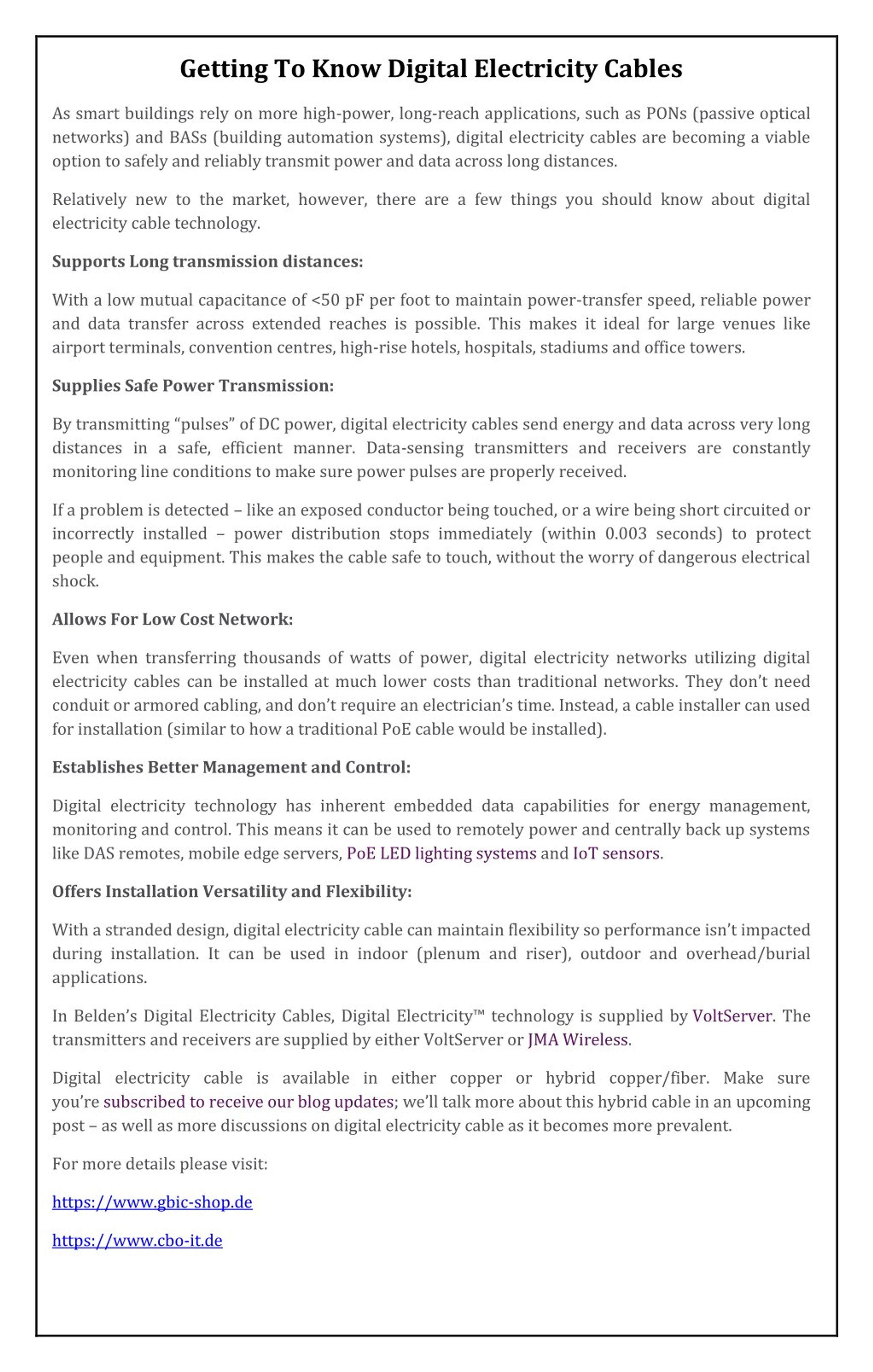This document, which appears to be a detailed guide or set of instructions possibly from an oracle or a similar source, is presented in a portrait orientation. It features a black border encompassing the entire layout. The main content is rendered in black font on a contrasting white background, with certain sections bolded for emphasis and some text appearing larger than others.

At the top center, the document is titled "Getting to Know Digital Electricity Cables," followed by two paragraphs that likely offer an introduction or synoptic overview of the topic.

Subsequently, a smaller bolded headline reads "Supports Long Transmission Distances," under which a warning is provided. Following this is another bold headline: "Supplies Safe Power Transmission," accompanied by two paragraphs elaborating on the safety aspects of power transmission.

The next section begins with a headline that states "Allows for Low-Cost Network." This is followed by a paragraph of information detailing how these cables facilitate low-cost networking. The text continues with information on "Establishes Better Management and Control," followed by an explanatory paragraph. This segment concludes with pink text that highlights "PoE LED Lighting Systems and IoT Sensors."

The final section is titled "Offers Installation Versatility and Flexibility," and it contains three paragraphs. In the second paragraph, there are hyperlinks associated with the terms "VoltServer" and "JMA Wireless," both marked in purple. The third paragraph includes bolded pink or purple text encouraging readers to "Subscribe to Receive Our Blog Updates."

At the bottom, the document directs readers to additional resources with the phrase "For more details, please visit," followed by two provided links.

This detailed layout ensures that the reader receives comprehensive information on digital electricity cables, inclusive of technical specifics, benefits, and additional learning resources.